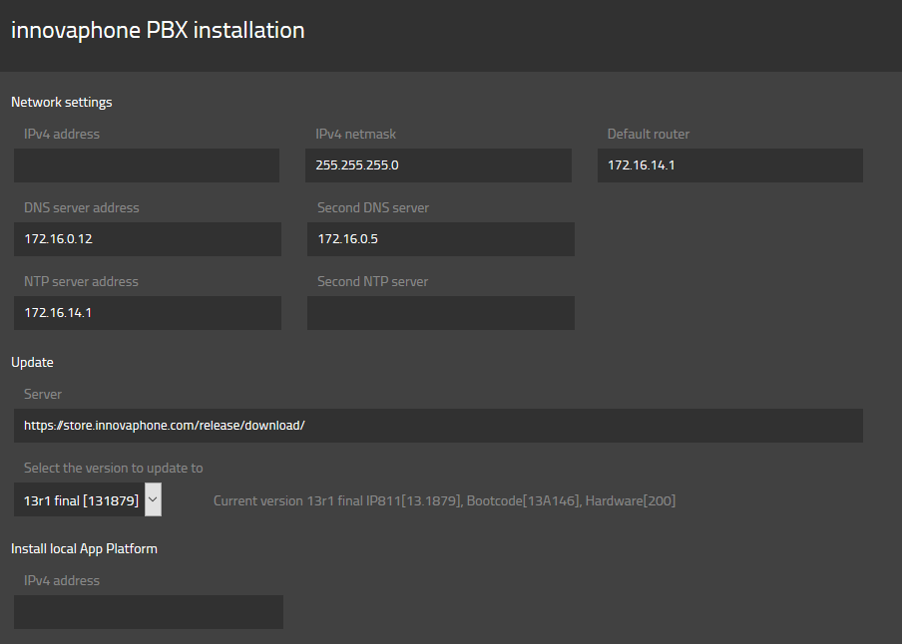A rectangular screenshot displays a menu box with a landscape orientation, resembling the dimensions of a landscape photo. At the top, a dark gray strip runs horizontally from left to right. In white, left-aligned text, it reads "InnovaPhone PBX Installation," with "InnovaPhone" spelled I-N-N-O-V-A-P-H-O-N-E and "PBX" in all caps.

Below the dark gray strip, the remaining lighter gray area contains various network settings details. The text elements within this section are:

- **Network Settings**
  - **IPv4 address:** (This field is currently blank)
  - **IPv4 netmask:** 255.255.255.0
  - **Default router:** 172.16.14.1
  - **DNS server address:** 172.16.0.12
  - **Second DNS server:** 172.16.0.5
  - **NTP server address:** 172.16.14.1
  - **Second NTP server:** (This field is currently blank)

Below these entries, the text "Update" appears, followed by:

- **Server URL:** https://store.innovaphone.com/.release/.download
- **Select the version to update to:** 13R1 final 131879.